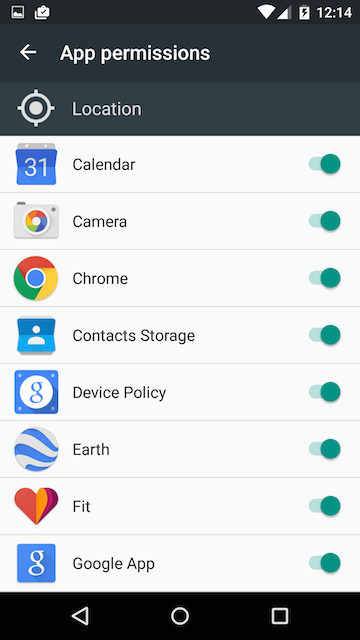The image displays a smartphone screen with its status bar showing the time as 12:14 PM and a thunderbolt symbol over the battery icon, indicating that the phone is currently charging. Below, there is a list of app permissions, each accompanied by a toggle switch. 

Here are the details of the image:
1. **Time and Charging Status**: The time is displayed as 12:14 PM, and there is a thunderbolt symbol over the battery icon, signifying that the phone is charging.
2. **App Permissions**: 
   - There is an arrow pointing to the left next to the list of app permissions.
   - Permissions shown include Location and Calendar.
   - All permissions have toggles that are switched on (the toggles are shaded, and the circles are aligned to the right).
   - Additional listed apps with their permissions switched on include Camera, Chrome, Contacts Storage, Device Policy, Earth, Fit, and the Google app.
3. **Navigation Bar**:
   - At the very bottom, there is a black rectangle which contains navigation icons:
      - A left-pointing white arrow.
      - A white circle.
      - A white square.

Overall, the image displays a smartphone screen with all the app permissions enabled and additional details on the charging status and navigation options.